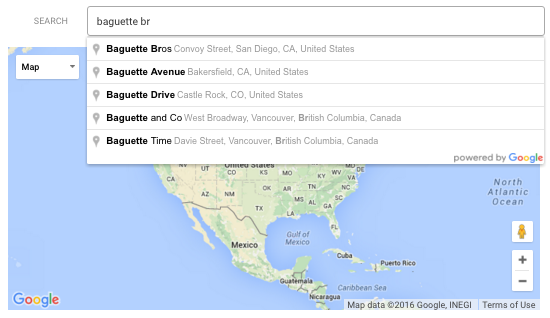Detailed Caption: 

The image shows a Google search interface for the term "baguette." In the upper-left corner, a gray text reads "Search." Below this, there is a white search bar with a gray outline, containing the text "B-A-G-U-E-T-T-E" followed by "B-R." Underneath the search bar is a list of search suggestions. These include:

1. **Baguette Bros** - Convoy Street, San Diego, California, USA.
2. **Baguette Avenue** - Bakersfield, California, USA.
3. **Baguette Drive** - Castle Rock, Colorado, USA.
4. **Baguette and Company** - West Broadway, Vancouver, British Columbia, Canada.
5. **Baguette Time** - Davie Street, Vancouver, British Columbia, Canada.

The font of the text is in either black or gray on a white background. In the bottom right corner of this section, it says "Powered by Google" in the characteristic Google colors: red, yellow, blue, and green.

Below these search suggestions, there is a map of North America prominently featuring the United States with parts of Mexico visible. The drop-down menu appears over much of the map. The Google logo appears in the left corner of the map in colors of blue, green, yellow, and black. 

In the upper-left corner of the map, there's a button labeled "Map" with an associated pull-down menu. In the bottom right corner, a yellow person icon is present within a white square, which is typically used for Google Street View. A plus and minus sign, each within white squares and connected, indicate map zoom controls. The North Atlantic Ocean is labeled in black font on the map.

At the very bottom right side of the image, a note reads: "Map data Copyright 2016 Google, INEGI, Terms of Use."